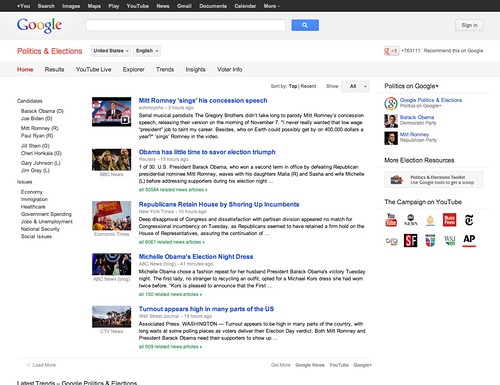Here is a polished and detailed caption for the given image:

---

Screenshot of the Google Politics and Elections webpage. At the top left corner, the header indicates "Politics and Elections." On the far left side, there is a list of candidates. Down the center of the page are five photographs, each accompanied by the headline of a related article. The right-hand side of the screenshot again references "Politics on Google Plus." Below this are various options, including circular icons and text that read "Google Politics and Elections," "Politics on Google Plus," "Barack Obama - Democrat," "Tech Party," "Mitt Romney - Republican Party," and "More Election Resources." Further down, there's a section titled "The Campaign on YouTube" featuring ten clickable icons representing different news organizations for additional reading.

---

This caption highlights all the key elements and their positions on the webpage, providing a clear and comprehensive description.